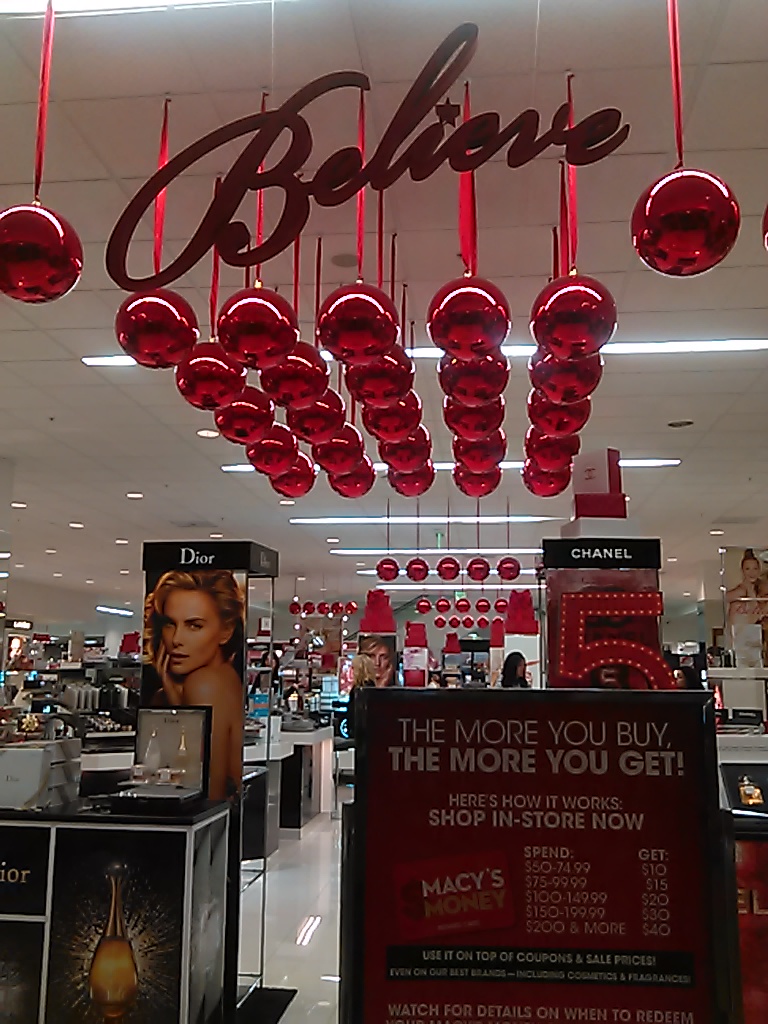Inside a bustling Macy's department store, the vibrant makeup section is adorned with festive decorations. Fluorescent lights hang from the white-tiled ceiling, illuminating the space. Red circular ornaments, resembling Christmas decorations, dangle from red strings, creating a cheerful, holiday atmosphere. A prominent, cursive "Believe" sign hangs from the ceiling, adding to the seasonal decor. The aisle is flanked by multiple display cases filled with cosmetics, including dedicated sections for renowned brands Dior and Chanel No. 5, each carefully enclosed and attractively presented. A large, red poster stating, "The more you buy, the more you get. Here's how it works: Shop in-store now at Macy's," prominently captures shopper’s attention with its enticing offer.